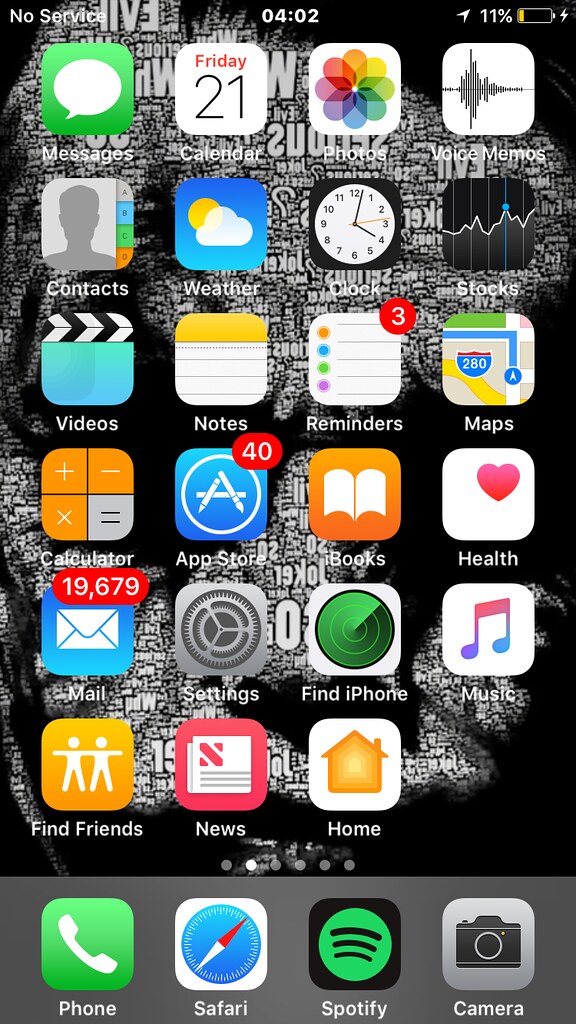A screenshot of an iPhone home screen features a unique wallpaper composed of various words arranged into abstract shapes. One discernible word, "Joker," is mirrored among others, forming an image that resembles a section of a map or globe, with land areas made up of these words.

From top to bottom and left to right, the iPhone displays standard apps including Messages, Calendar, Photos, Voice Memos, Contacts, Weather, Clock, Stocks, Videos, Notes, Reminders (with three notifications), Calculator, App Store (with 40 notifications), Books, Health, Mail (with 19,679 notifications), Settings, Find iPhone, Music, Find Friends, News, and Home. At the bottom dock, customized apps include Phone, Safari, Spotify, and Camera.

The phone shows the time as 16:02 in 24-hour format, has a battery life at 11%, is currently charging, has no service, and location services are enabled.